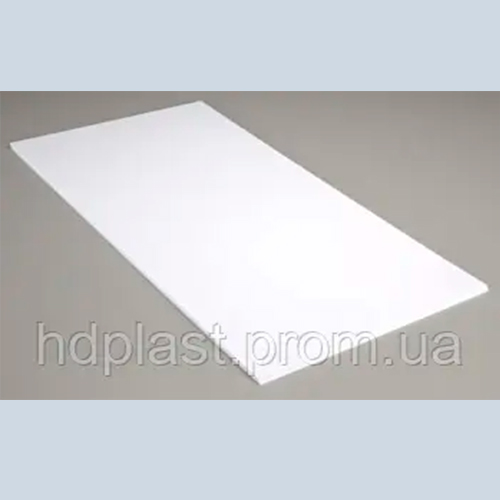The image is a perfectly squared composition featuring a prominently letterboxed style with light blue-gray bars spanning the top and bottom. The central background is a medium brown, reminiscent of a ground surface, while a pristine white rectangle lies diagonally from the upper left to the lower right, simulating a yoga mat. Overlaying the bottom of this brown section, and extending across the "mat," is semi-transparent white text with a 3D effect that reads "hdplast.prom.ua." Dominating the color scheme are shades of light blue, gray, white, and brown, creating a visually striking and minimalist geometric design.